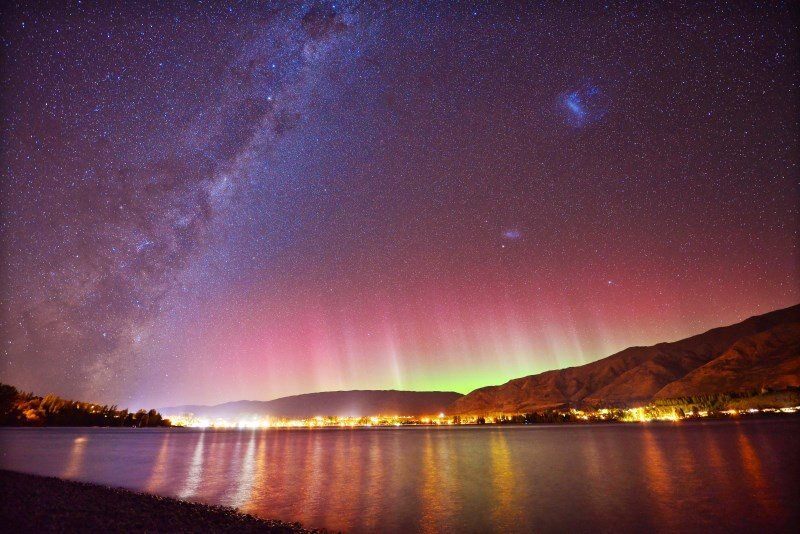The image captures a stunning outdoor nighttime scene featuring a mesmerizing display of the Aurora Borealis. The sky, a deep dark purple gradient transitioning to pink and yellow, is sprinkled with countless glittering stars that lend a sense of magic to the landscape. On the left side, mysterious billowing clouds or swirls add depth and intrigue. In the foreground, rolling brown hills and mountains frame a quaint town below, its warm lights casting a welcoming glow. This town nestles along the shore of a serene lake, which mirrors the vibrant hues of the northern lights and the myriad stars above. The aurora's colors range spectacularly from neon yellows and whites to rich pinks, greens, reds, oranges, and purples, creating an awe-inspiring contrast against the darkened, starry sky. The reflection in the lake captures this celestial spectacle as well as the cozy lights from the town, making the scene appear almost dreamlike.